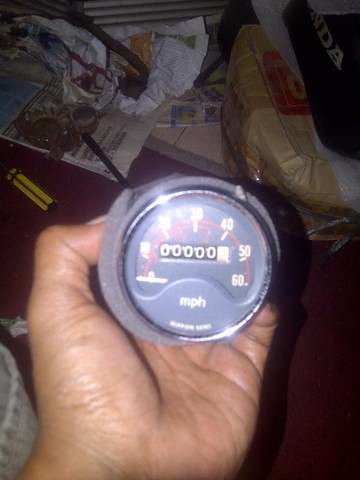In this image, a person’s hand is prominently featured at the bottom, holding a circular, gray object reminiscent of a speedometer or timer. The object has a glass front, revealing a display underneath that bears a striking resemblance to a speedometer. The display features numerals increasing in increments of ten (10, 20, 30, 40, 50, 60), arranged in a semi-circular pattern. These numerals are white and are accompanied by a red arc that traces their path. Beneath the semi-circle of numbers, there's a white rectangular section displaying "0000" in white digits. At the bottom of the circular display, the abbreviation "MPH" is visible in white letters, with smaller, less legible white text underneath it.

The hand holding this object is positioned against a maroon background that appears to be a bed sheet. In the upper part of the image, various miscellaneous items are scattered. There are crumpled and flattened papers, possibly newspapers, with coins scattered on top of them. A yellow-handled screwdriver also lies amidst this array on the maroon bedding. Additionally, an old, small box, taped up and seemingly filled with assorted items, is visible, contributing to the cluttered scene. All these elements together create a sense of casual disarray within the setting.